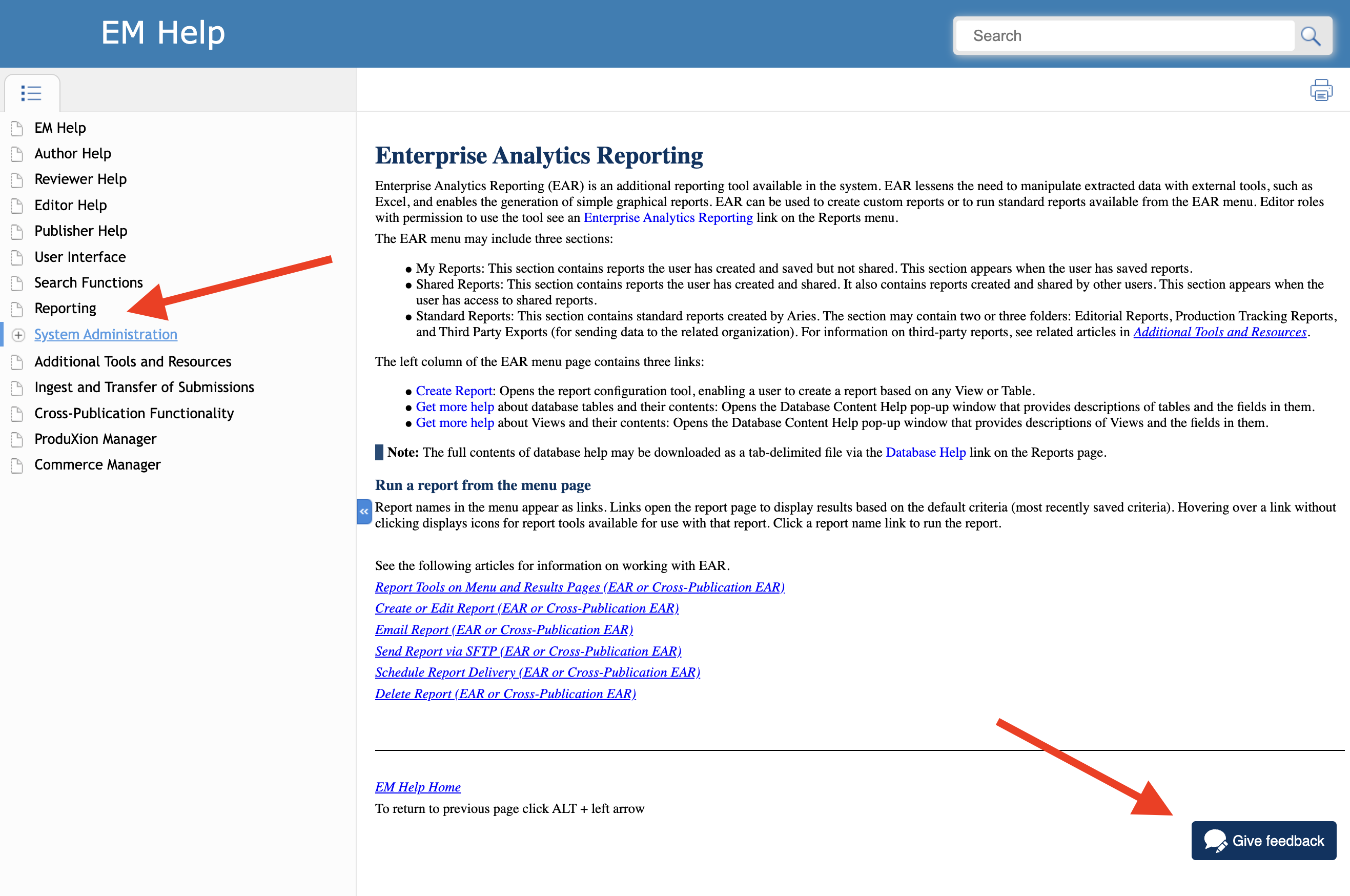This screenshot captures the interface of a help page on a website. The top section features a blue banner with the text "EM Help" prominently displayed in white letters. To the right of the banner, there is a search bar.

The main body of the screenshot is divided into two sections. On the left side, there is a menu with various help options, listed in the following order: Exit Help, EM Help, Author Help, Reviewer Help, Editor Help, Publisher Help, User Interface, Search Functions, and Reporting. A red arrow has been added to the page, pointing directly at the "Reporting" option.

On the right side of the screenshot, the content related to the selected "Reporting" option is displayed. The heading reads "Enterprise Analytics Reporting," followed by detailed information pertaining to this topic. Another red arrow on the page is angled downwards toward the bottom right corner, directing attention to a "Give Feedback" button.

Overall, the screenshot has been edited to guide users through the process of selecting "Reporting" from the help options and then clicking on the "Give Feedback" button. The background of the website is white, ensuring that the text and elements are clearly visible.